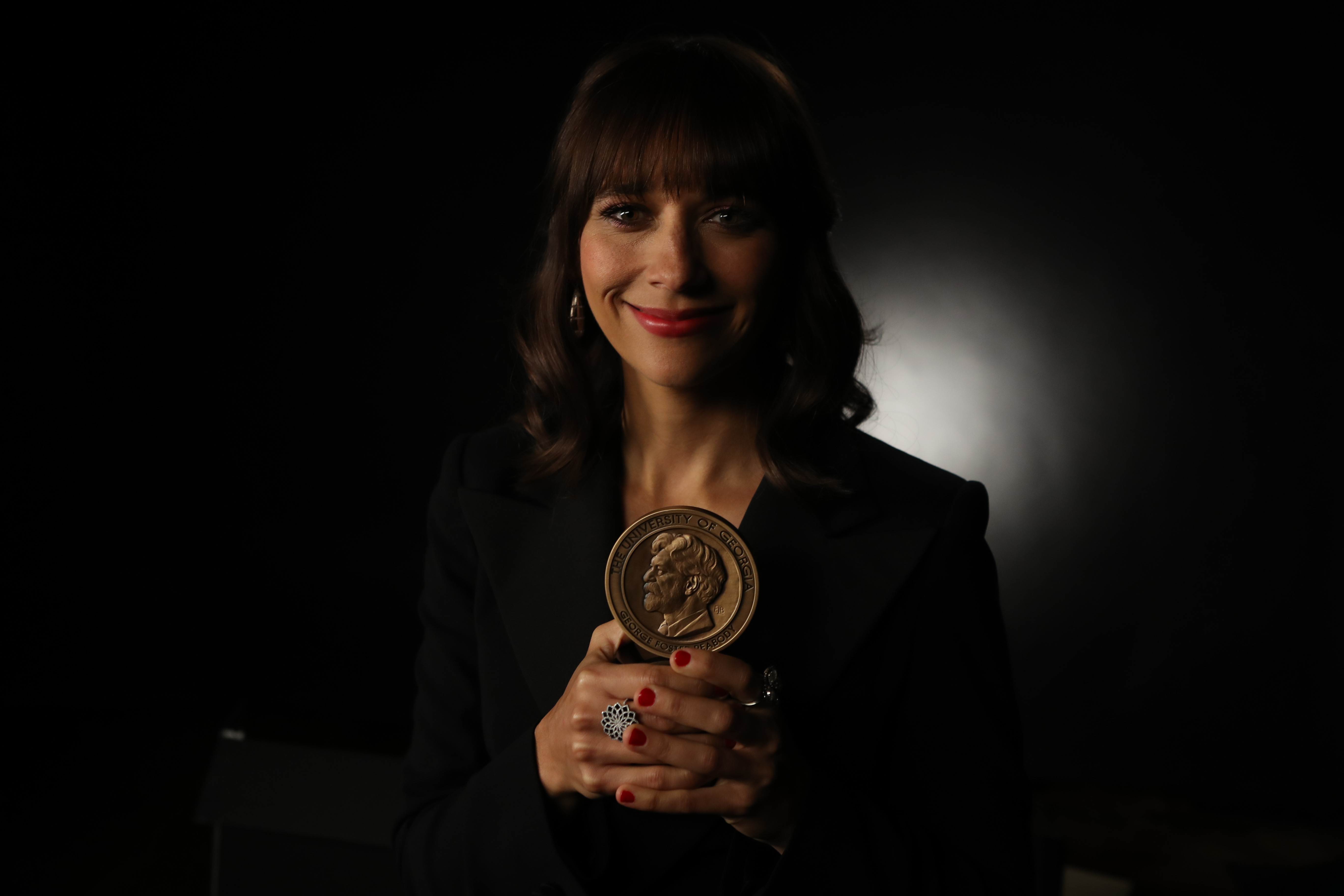The close-up image features Rashida Jones centered against a nearly entirely black background, with a faint hint of white light visible over her right shoulder. Rashida has shoulder-length, brown, curly hair with bangs and tan skin. She is wearing red lipstick and makeup around her brown eyes, which accentuate her smile, although her teeth are not shown. Hoop earrings can be seen peeking out from her curly locks. She is dressed in a black suit jacket that blends seamlessly into the dark background. Her hands are positioned in front of her, showcasing red nail polish and a flower ring while holding an award—a large coin or medal that depicts the profile of an older man with medium-length hair and a goatee, emblazoned with the "University of Georgia."